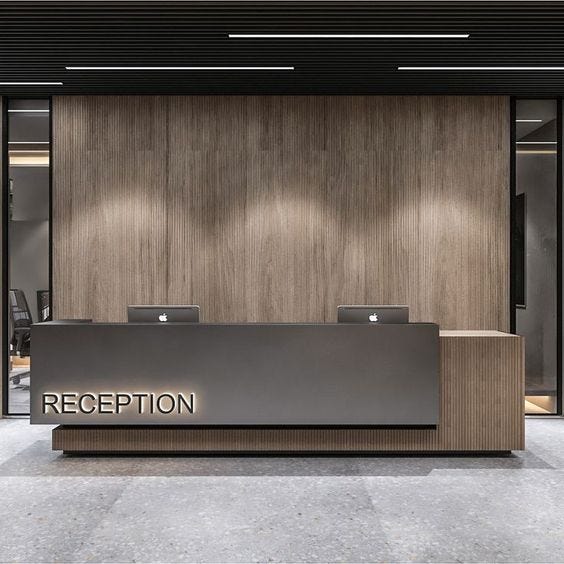The image depicts a clean and refined corporate lobby area. The focal point is a large reception desk situated in the center. The desk features vertical brown and gray lines with a smooth gray top section, and the word "reception" is prominently displayed in dark letters that glow with a white backlight. Two Apple computers, identifiable by their logos, are positioned at each end of the desk. Behind the reception area, there is a floor-to-ceiling wall adorned in dark brown wood grain paneling. On either side of the desk, glass windows provide a view into adjacent rooms. The left window reveals a meeting room with modern business chairs, while the right window hints at a space with a blackboard. Overhead, the ceiling is black with thin white lights, and the floor is made of large, smooth, gray granite tiles, contributing to the polished and professional ambiance of the space.